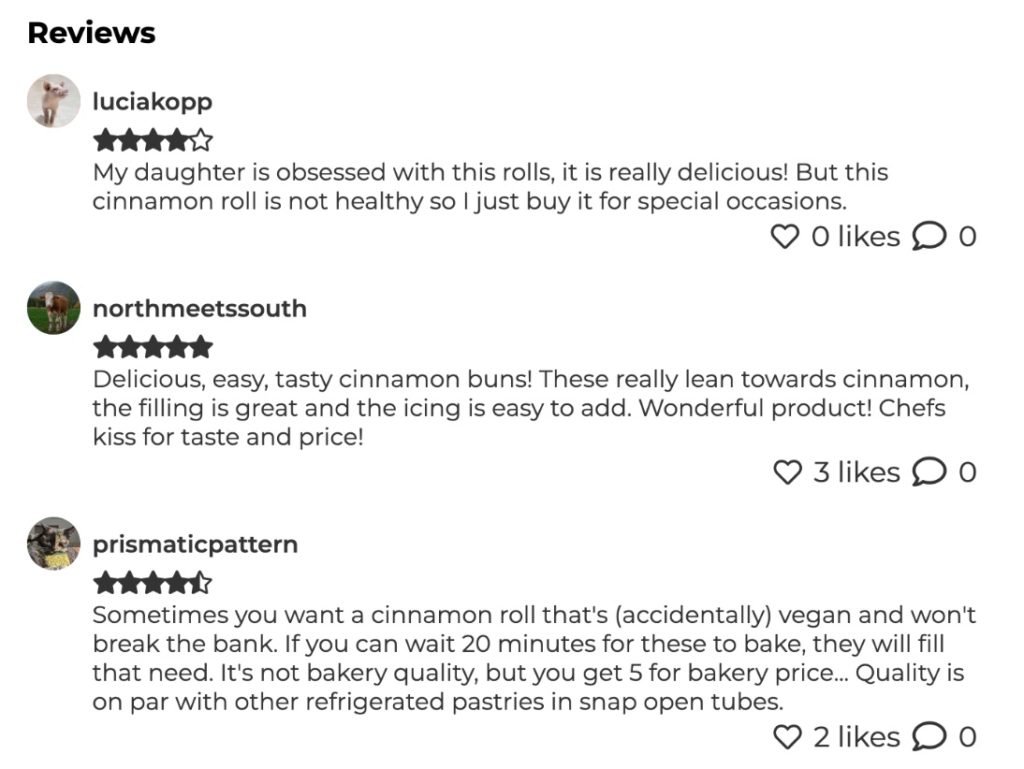This image is a screenshot of a review section from an online platform. The background is white, and the top left corner features the word "Reviews" in bold black text. Below this heading are three user reviews, each accompanied by a small circular user profile picture.

**First Review:**
- **User:** Lucia Cop
- **Rating:** 4 out of 5 stars
- **Comment:** "My daughter is obsessed with these rolls. They are really delicious, but this cinnamon roll is not healthy, so I only buy it for special occasions."

**Second Review:**
- **User:** NorthMeetSouth
- **Rating:** 5 out of 5 stars
- **Comment:** "Delicious, easy, tasty cinnamon buns. These really lean towards cinnamon. The filling is great, and the icing is easy to add. Wonderful product. Chef's kiss for taste and price."

**Third Review:**
- **User:** Prismatic Pattern
- **Rating:** 4.5 out of 5 stars
- **Comment:** "Sometimes you want a cinnamon roll that's accidentally vegan and won't break the bank. If you can wait 20 minutes for these to bake, they will fill that need. It's not bakery quality, but you get five for bakery price. Quality is on par with other refrigerated pastries in snap-open tubes."

Each review offers a distinct perspective on the product, with detailed notes on taste, convenience, and value.